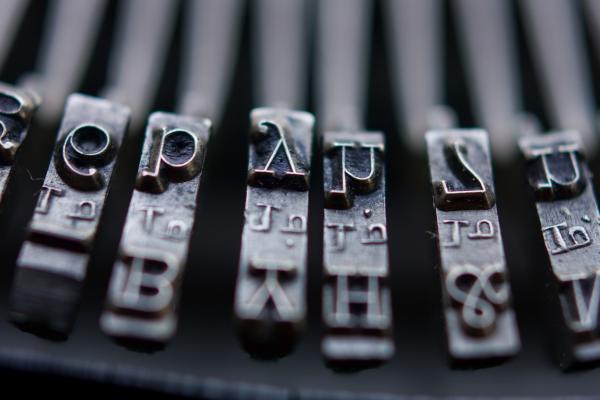The image captures a close-up of what appears to be metal typewriter keys, set against a blurred gray background. The keys are oriented with their embossed letters upside down, creating a distinct, detailed forefront. Each key features a prominent Greek letter at the top, followed by the letters 'JN' or 'IN' with dots positioned variably—above, below, or beside the 'N.' Some letters appear to be mirrored or rotated, such as a backward 'E,' a 'P,' an upside-down 'Y,' and a backward 'Y.' The lower portions of the keys also bear additional Greek letters, including an upside-down '7' and a 'U.' Portrait mode in the photograph makes the metal keys clear and pronounced, though the extending parts behind them are blurred and indistinct, suggesting they are part of a larger mechanism. The metal structure gleams subtly, emphasizing the precision of the engraved letters and the complex arrangement of dots and symbols.